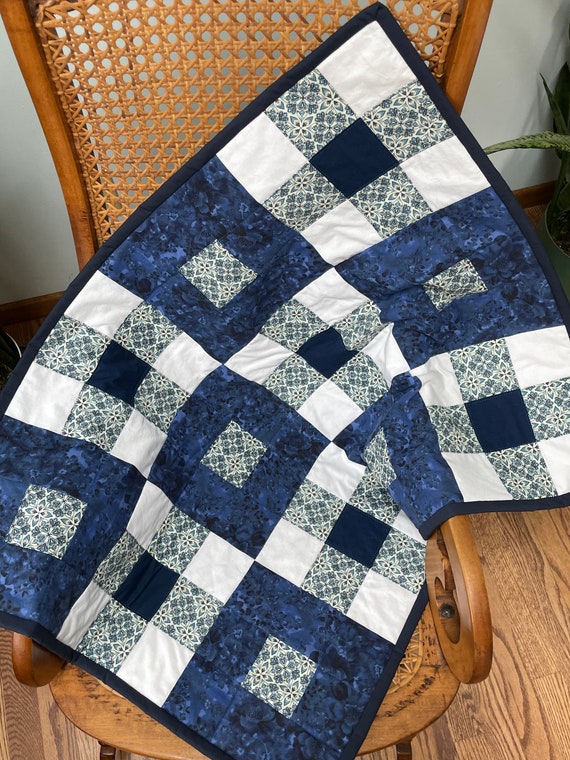In the image, we see a brown wooden chair with its seat and backrest crafted from a net-like, wicker material. Draped over the chair is a distinctively patterned, multicolored blanket. This blanket predominantly features a checkerboard pattern composed of alternating blue, white, and gray squares. The blue squares each contain nine smaller squares with a central gray dot, while the white squares have a black dot in the center, flanked by gray atop and below. The border of the blanket is a dark blue, which gently contrasts with the lighter shades within the squares. The wooden floor beneath the chair is similarly brown, complementing the color palette. In the background, a gray wall can be seen, and in the top right corner of the frame, a part of a green plant with a few leaves adds a touch of natural detail. This photo appears to be taken indoors with a vantage point looking down at the chair and blanket, highlighting the meticulous design and texture present in both the chair's wicker construction and the blanket's intricate pattern.